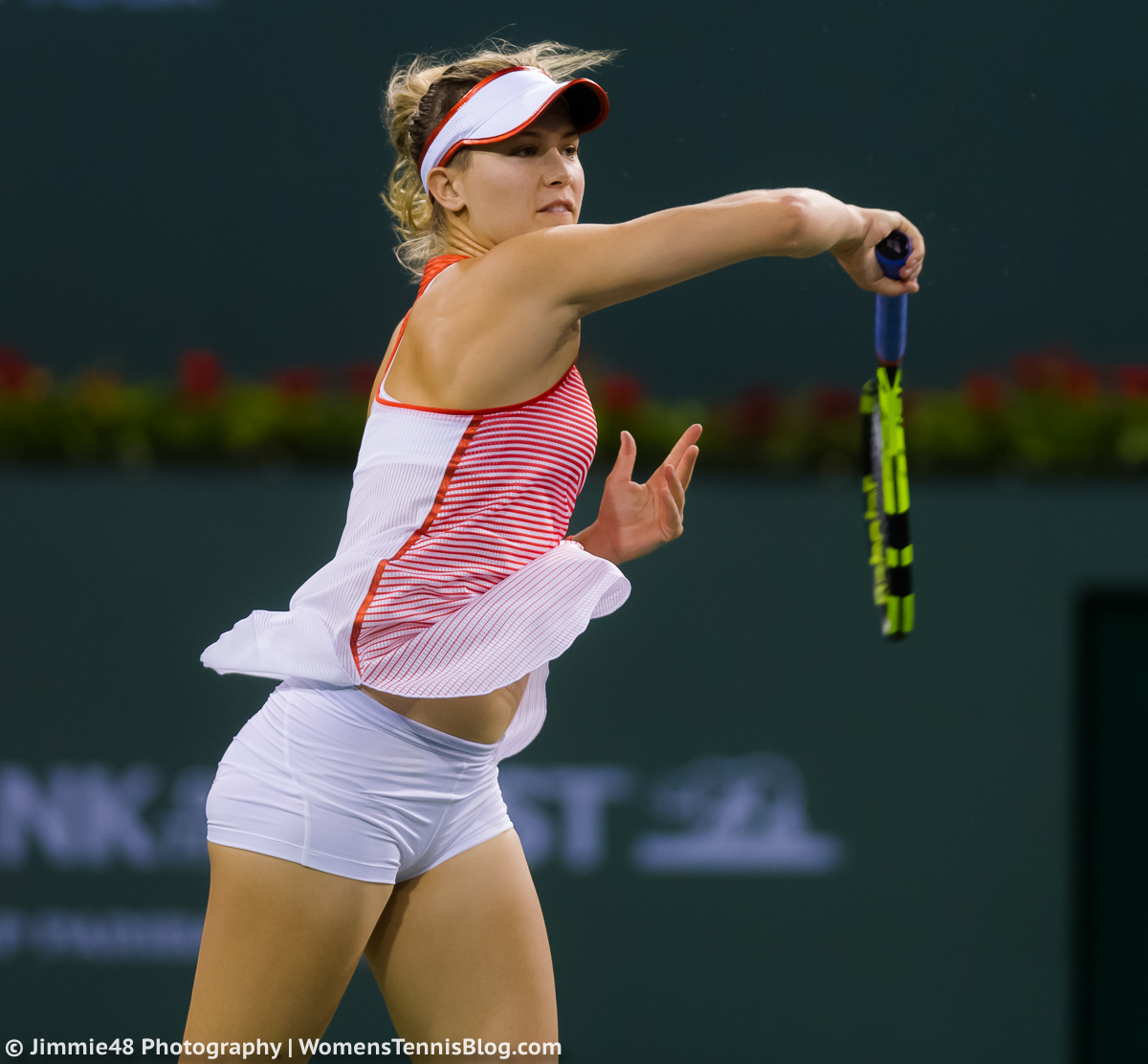This photo captures tennis player Eugenie Bouchard in the midst of an intense match. She is swinging her blue, yellow, and black racket with her right hand, her left hand extended out to the side. She is dressed in a white and red sun visor that holds back her blonde hair, which is tied in a ponytail swaying with her movement. Her outfit consists of a loose tank top with red and white stripes on the front and white on the back, billowing upward due to her fast motion, revealing her almost skin-tight, very short white shorts. The scene is set against an out-of-focus background featuring a dark gray tennis wall with indistinct sponsor logos. At the bottom left corner of the image, there is white text that reads "Copyright Jimmy48Photography/Women'sTennisBlog.com."